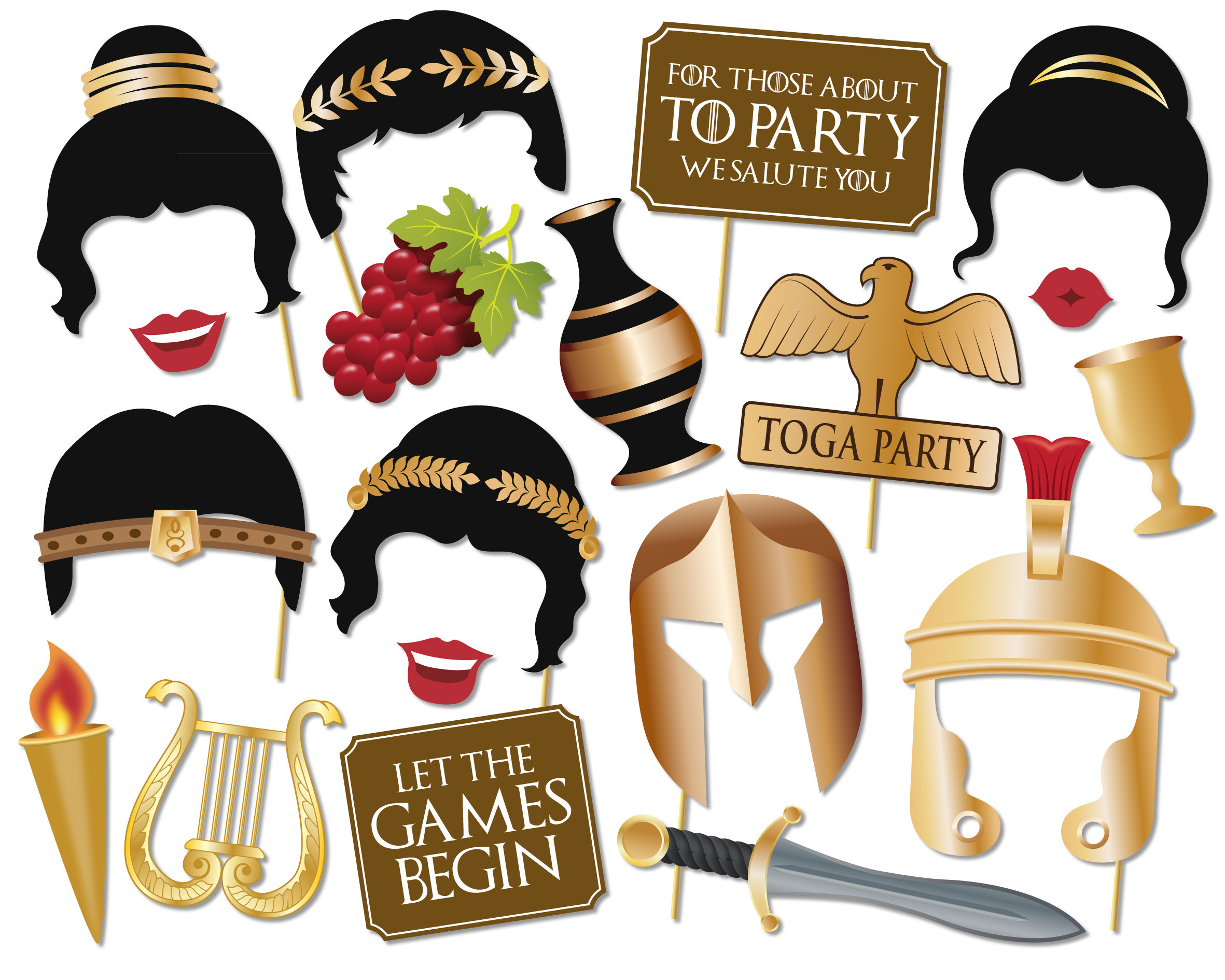The image is a richly detailed collection of vector art illustrations, predominantly featuring stylized representations of heads with distinct hairstyles and accessories. The illustrations are designed to resemble masks or stickers that can be used for character creation or artistic projects. Prominently, there are several silhouettes of female heads with black hair, some adorned with gold items and red lipstick, and others styled into elegant buns wrapped in gold.

In addition to the female figures, there are representations of male heads characterized by black hair and often crowned with gold wreaths or Roman guard helmets. The scene is punctuated by various thematic elements such as gold knight helmets, an ornate gold chalice, an eagle, a lit and burning torch, and a black vase with gold accents. Musical instruments like a harp, as well as regal and celebratory symbols such as swords and grapes, add to the richness of the collection.

Scattered among the illustrations are three brown signs with white text. The top right sign reads, "For those about to party, we salute you," while another indicates "Toga party" with a bird symbol atop it. The bottom left corner features a sign that says, "Let the games begin." The entire setup evokes a festive and adventurous spirit, suggestive of a grand toga-themed celebration, blending elements of ancient Roman and Greek iconography for an artistic and playful visual experience.